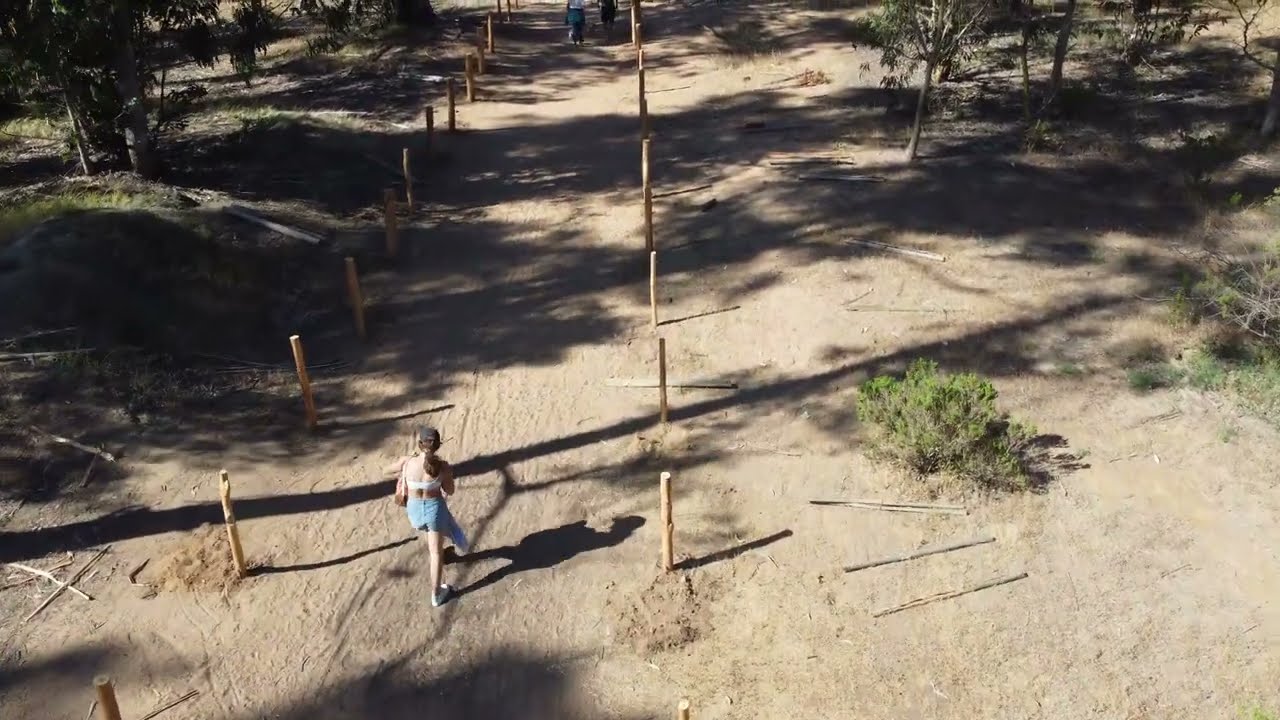This overhead photograph captures a woman walking along a straight, brown dirt road flanked by wooden posts. The scene is set in a forested area with trees and patches of green grass on both sides of the path. The woman, centrally positioned in the image, has long brown hair tied in a ponytail and wears a black or gray baseball cap. Her outfit consists of blue denim shorts, a white top or bra, and white sneakers. She carries a purse on her left shoulder and has her back facing the camera. Further ahead on the trail, there are two figures walking, their heads partially out of frame. The image is suffused with daylight, casting shadows from the surrounding trees.